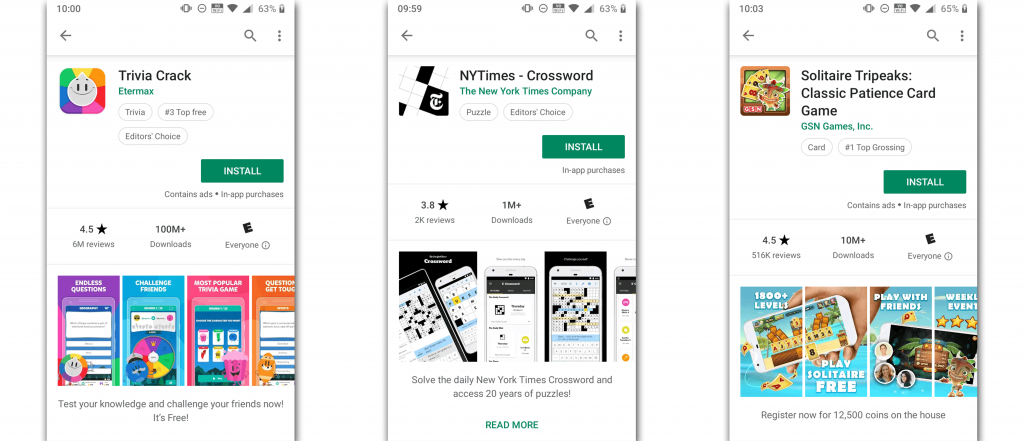This image features three screens, displayed side-by-side: one on the left, one in the center, and one on the right. 

**Left Screen:**
At the top left of this screen, the time is displayed as "10:00". To the right of the time, several icons are visible, albeit small and difficult to identify. Noteworthy icons include:
- A vibrate icon
- A Wi-Fi icon
- A cellular network icon
- A battery icon with a charge level of 62%

Below the status bar, the screen showcases the app "Trivia Crack", spelled "TRIVIA crack". Underneath this app name, it reads "Etermax", spelled "E-T-E-R-M-A-X". There are several tabs below this, including:
- "Trivia"
- "Top Free" marked as number three
- "Editor's Choice"

On the left side of this app display, the app's logo is prominent. The logo features a smiling face centered amidst a vibrant, multicolored background. The colors visible in the backdrop are blue, green, yellow, red, pink, purple, and orange.